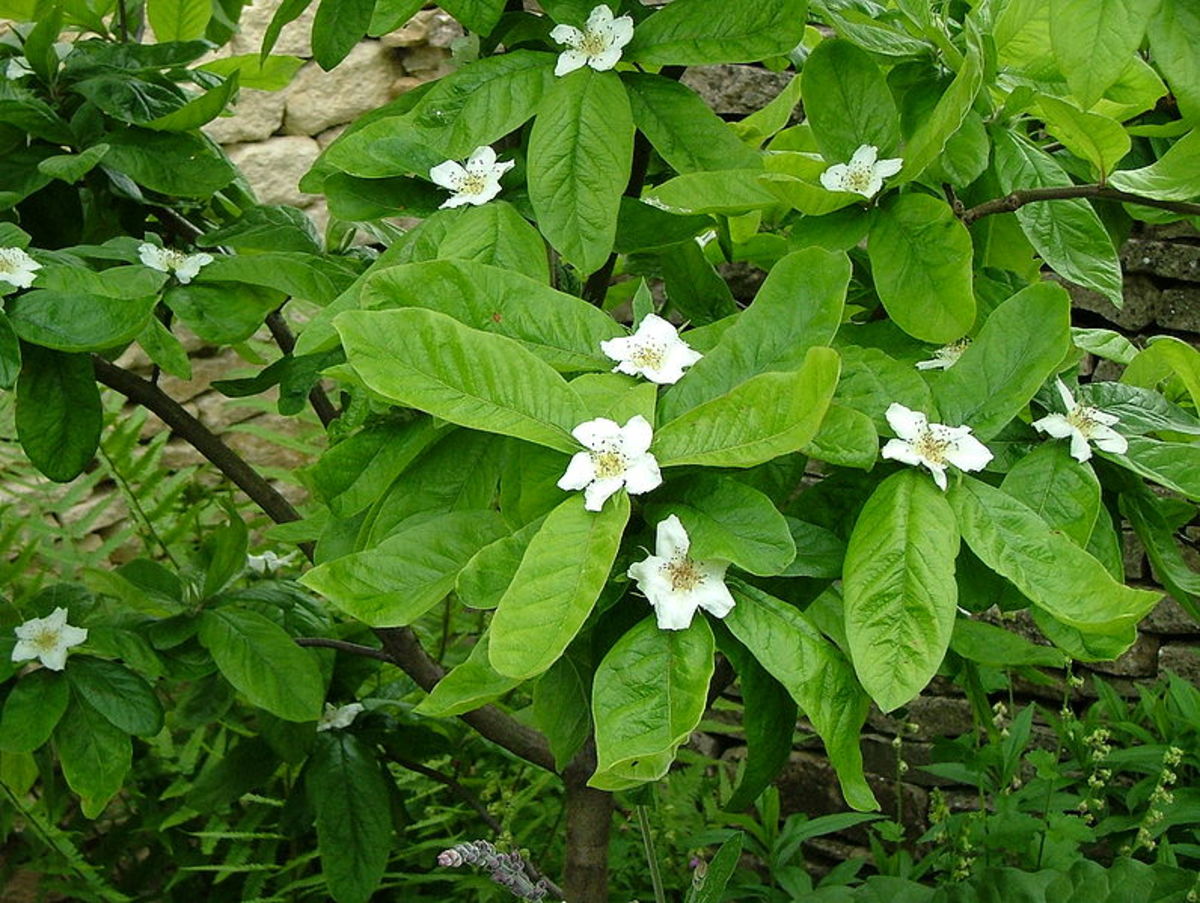This photograph captures a lush, green bush in full bloom, set against a stone-layered wall. The bush boasts bright green, elongated leaves, each approximately five inches in length, radiating from its woody stems. Nestled among the leaves, small, dainty white flowers with five petals each showcase detailed, prominent pistils. The centers of the flowers are a striking yellow, dotted with black. The image is brightly focused in the middle, highlighting the vivid colors and intricate details of the flowers and leaves, while the background softly blurs, hinting at fern fronds and emphasizing the bush against the stone wall. The outer edges of the photograph are darker, drawing attention towards the sunlit, vibrant center of the image. This composition suggests an outdoor setting, possibly taken on a cloudy day, and conveys a sense of natural beauty and detailed botanical structure.